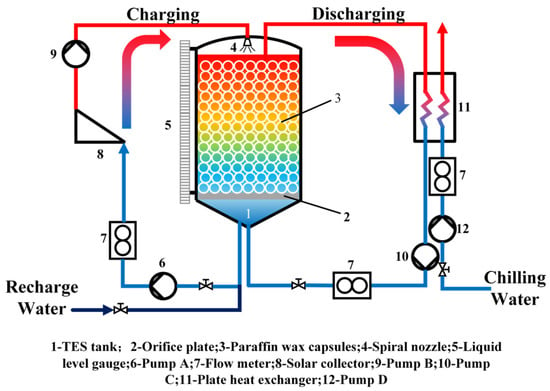This detailed diagram depicts a color-coded system related to the processes of charging and discharging water and energy. At the top, in black text, the headings "charging" on the left and "discharging" on the right frame a central, multicolored, pentagonal graphic which exhibits a gradient transitioning from red at the top, through yellow and green, to blue at the bottom. This gradient is marked by a series of red, purple, and blue arrows.

The diagram is divided into sections, with "recharge water" indicated at the bottom left and "chilling water" at the bottom right. Additionally, the diagram is annotated with several numbers (9, 8, 5, 4, 3, 2, 6, 7, 10, 12, 7, and 11) that correspond to a comprehensive list of components at the very bottom of the image. These components are detailed as follows:

1. TES tank
2. Orifice plate
3. Paraffin wax capsules
4. Spiral nozzles
5. Liquid level gauge
6. Pump A
7. Flow meter
8. Solar collector
9. Pump B
10. Pump C
11. Plate heat exchanger
12. Pump D.

This structured and colorful visual tool serves to illustrate the complex interplay of these components within the water and energy system.